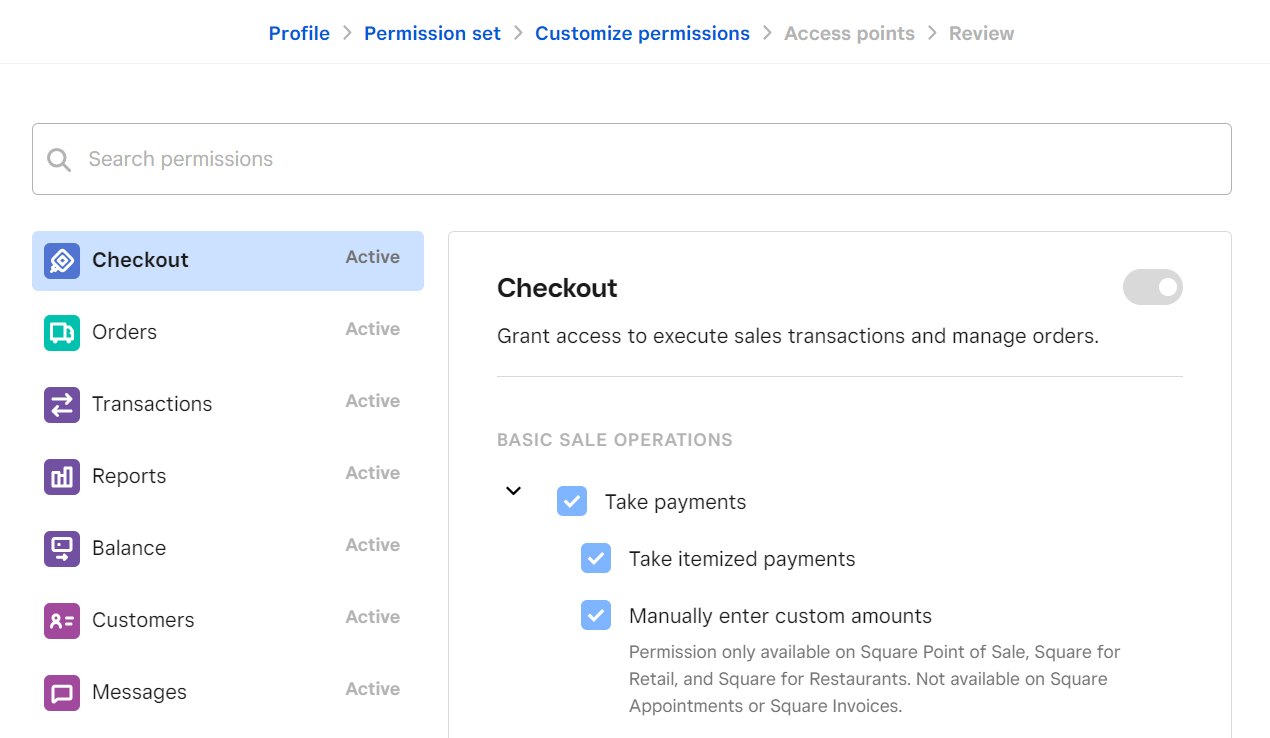This image depicts a settings page for a website with a clean and organized layout. The background is white, adorned with dark gray or black text, medium gray text for less prominent information, and blue links for navigational elements. On the left side of the page, there is a vertical menu accompanied by matching icons that guide users through various settings options. The icons transition through a gradient of colors—blue, green, and purple down to red, except for the green icon for 'Orders,' which stands out.

At the top, the header features breadcrumb navigation links, providing a clear path to the user’s current location within different levels and categories of settings. Below the header, there is a search bar displaying the placeholder text 'Search permissions,' making it easy for users to find specific permission settings.

The left-hand menu includes options such as 'Check out,' 'Orders,' 'Transactions,' 'Reports,' 'Balance,' 'Customers,' and 'Messages.' Each option is active and has a corresponding icon. The 'Check out' section has a green icon and features a description to the right that states, "Grant access to executive sales transactions and manage orders." This option is currently toggled off.

Underneath, the 'Basic Sales Operations' section includes a list of checkboxes, all checked, with options like 'Make payments,' 'Make itemized payments,' and 'Manually enter custom amounts,' each accompanied by explanatory text for further clarification. The detailed and structured layout ensures the settings page is user-friendly and intuitive, facilitating seamless navigation and comprehension.